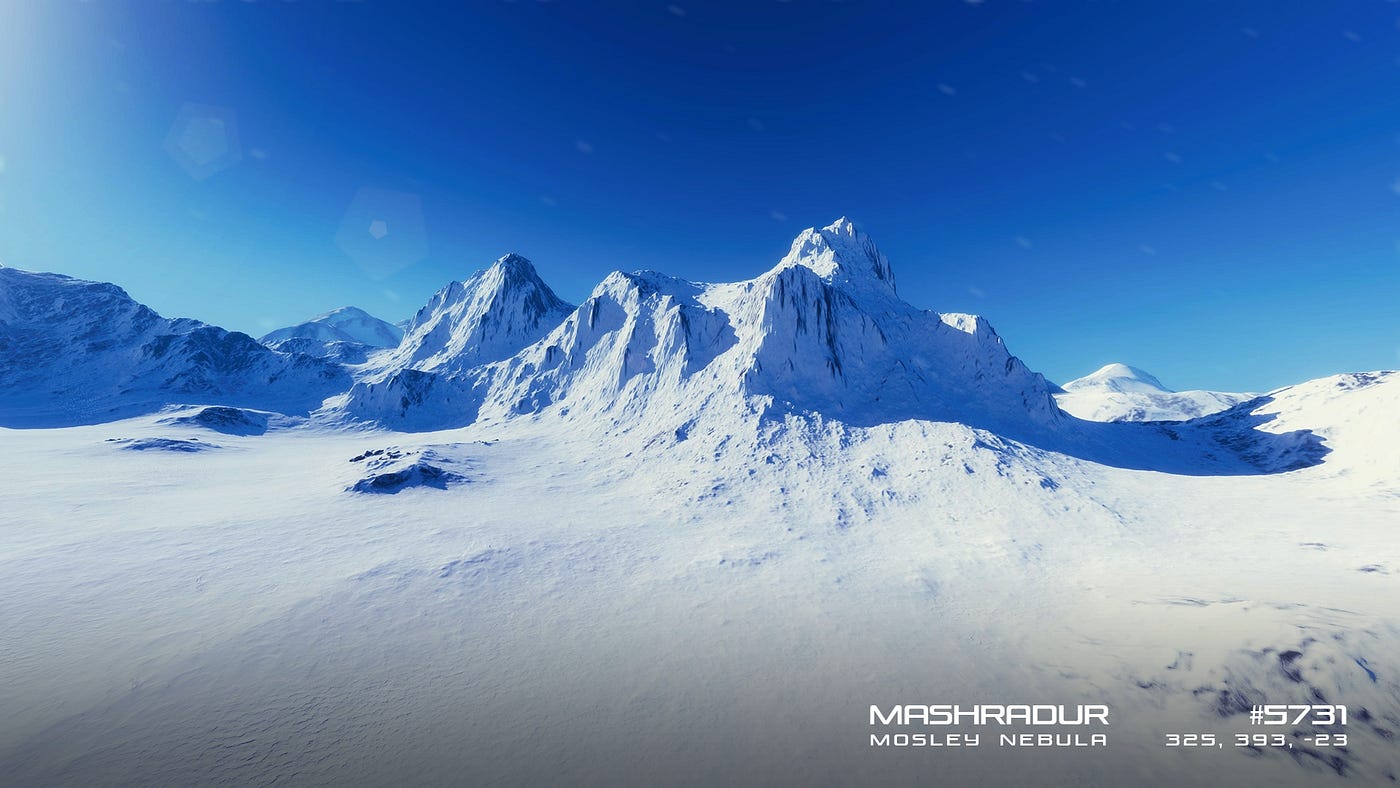The photograph captures a pristine winter landscape dominated by a lone, craggy mountaintop. The scene is bathed in bright sunlight, with the sun positioned to the left, casting long shadows to the right across the untouched white expanse of snow. The sky above transitions from light to medium blue, creating a striking contrast against the immaculate white and gray hues of the snowy and rocky mountain. No footprints or signs of human presence are visible, emphasizing the remote and untouched nature of the setting. In the background, slightly out of focus, additional mountains can be seen, adding depth to the image. The only text in the photograph is located in the lower right corner, reading "Mash-R-Dur, Moseley Nebula," followed by the coordinates "5731, 325.393-23." The stark beauty and isolation of this icy, snowy environment suggest it could be from a remote area like Antarctica or Siberia.